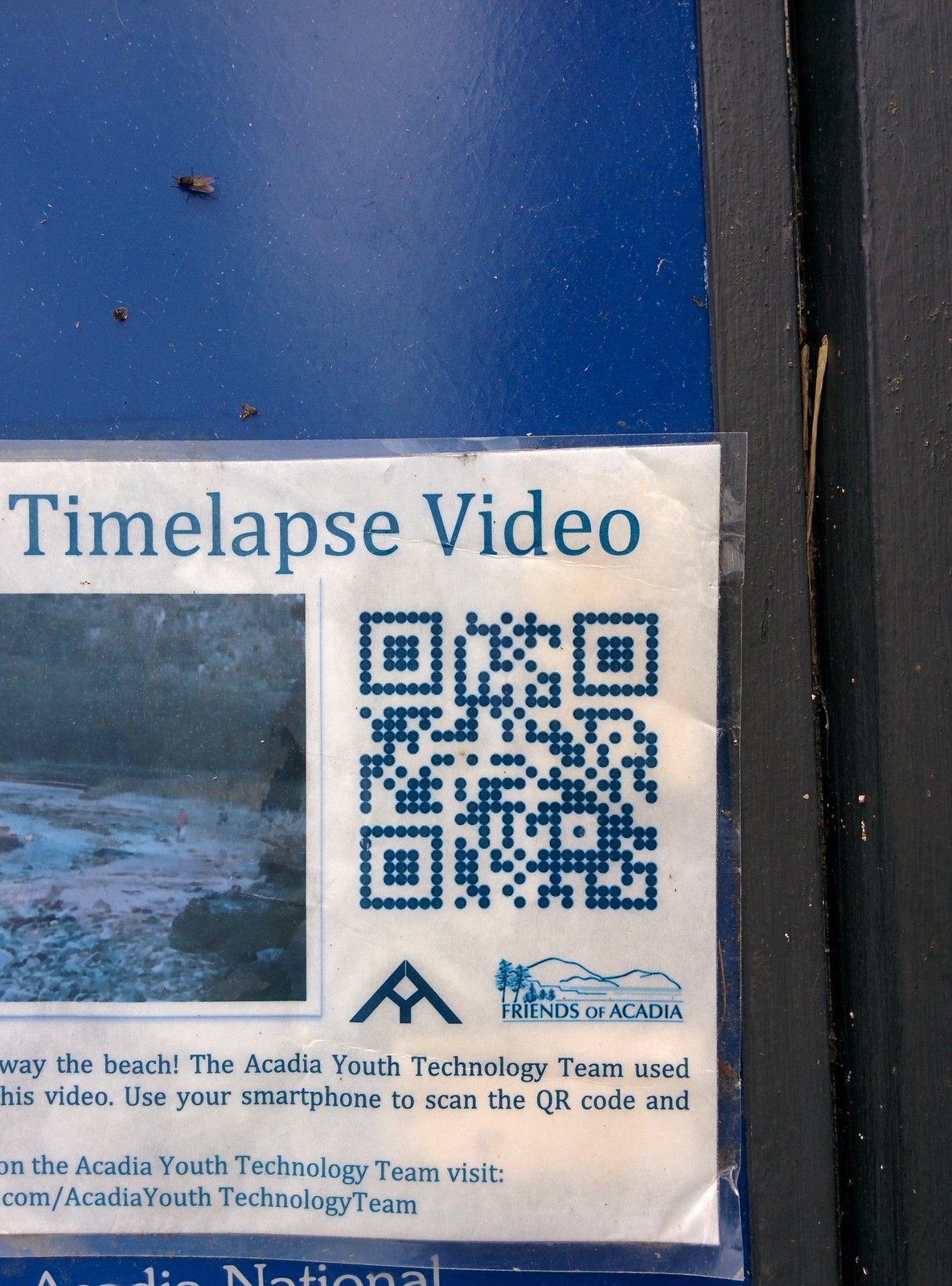The image displays a close-up photo of a notice that’s taped to what seems to be an outdoor blue wall or door. The title of the notice reads "Time Lapse Video," though part of the text on the left side is cut off, making it partially unreadable. Below the title, there is a partially visible landscape photo, seemingly a stream with numerous rocks. Beneath the word “Video,” a QR code is printed next to the logo for "Friends of Acadia." The accompanying text mentions the Acadia Youth Technology Team and provides a URL to a website, along with instructions to use your smartphone to scan the QR code for more information. The poster is situated towards the bottom of the image, and in the upper part of the image, a fly is visible on the wall. The color scheme includes shades of blue, gray, and hints of brown and orange.